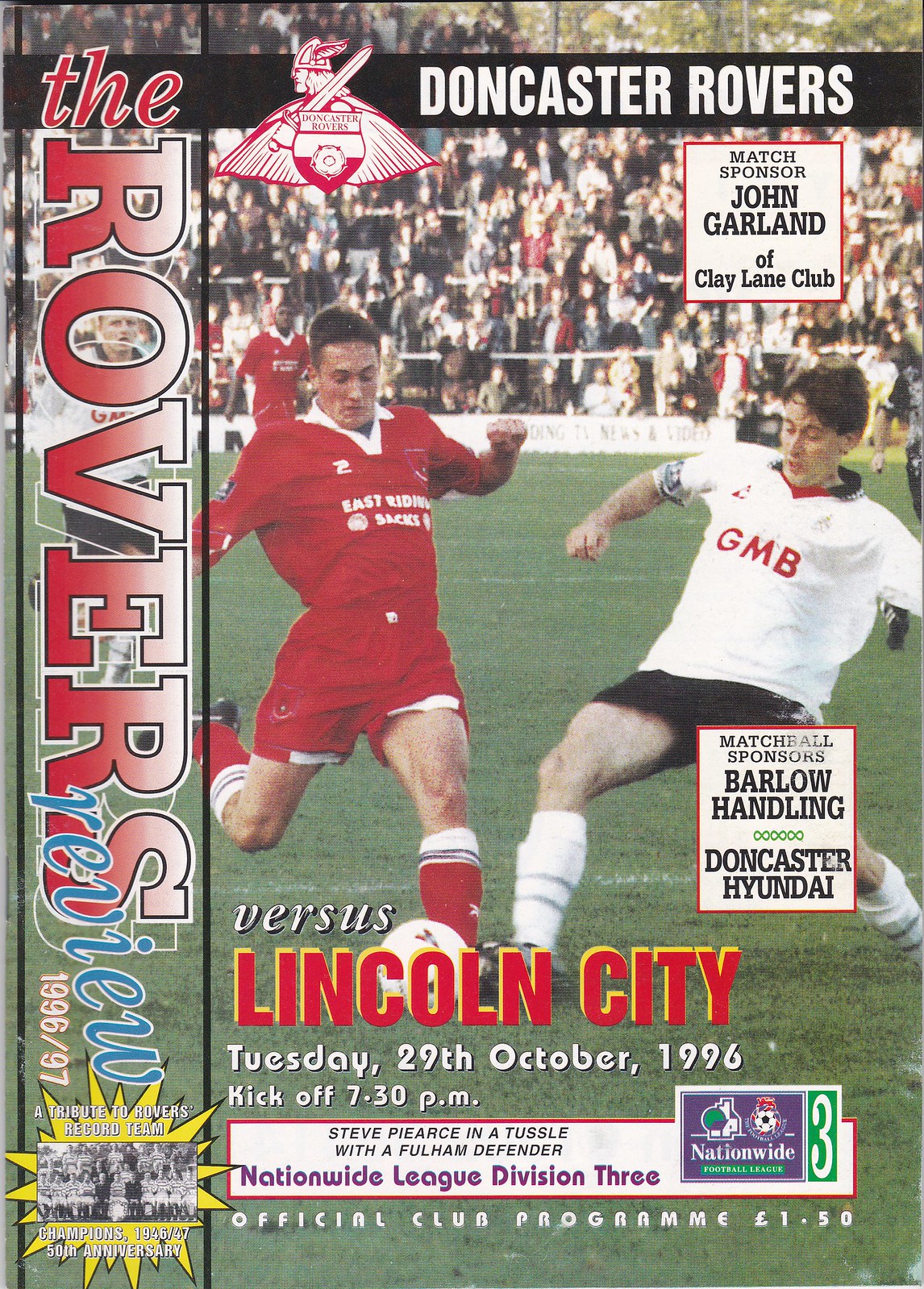A vibrant scene from a sports program for a soccer match captures the intensity of the competition. In the background, an enthusiastic crowd adds to the electrifying atmosphere. In the foreground, two players are locked in a fierce battle for the ball. On the left stands a player dressed entirely in red, his expression focused and determined. On the right, his opponent, wearing a white shirt emblazoned with "GMB" and dark shorts, mirrors his intensity. This image represents the match between the Rovers and Lincoln City, held on Tuesday, October 29th, 1996, with a kickoff at 7:30 PM. The program marks this event as a significant English soccer match.